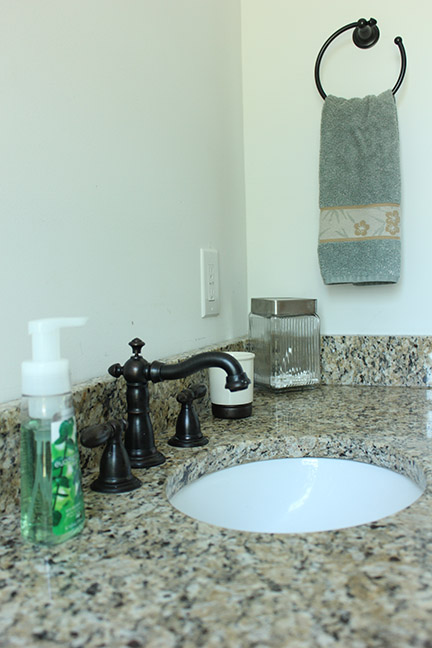The photo captures a meticulously clean and well-organized bathroom sink area, showcasing a luxurious marble countertop. The countertop features a beige base with specks of black and white, giving it a distinctive speckled marble appearance. Centrally placed in the countertop is a white sink, framed by the same marble material. The faucet, described as resembling a tall, brown pepper shaker with a pull-up button, is elegantly curved and delivers water through two small spouts, one for hot water and one for cold, positioned on either side.

To the right of the sink, there is a small, white cup with a brown base, likely intended for toothbrushes or mouthwash. Adjacent to this, a glass container with a tin lid holds neatly arranged cotton swabs. An electrical outlet is visible above the counter on a white-beige wall. Mounted on this wall to the right is a hook holding a face towel or hand towel. The towel is primarily light gray to light blue with a decorative strip featuring yellow flowers on a beige background. On the left side of the countertop, there's a green soap bar adorned with a floral design, completing the scene.